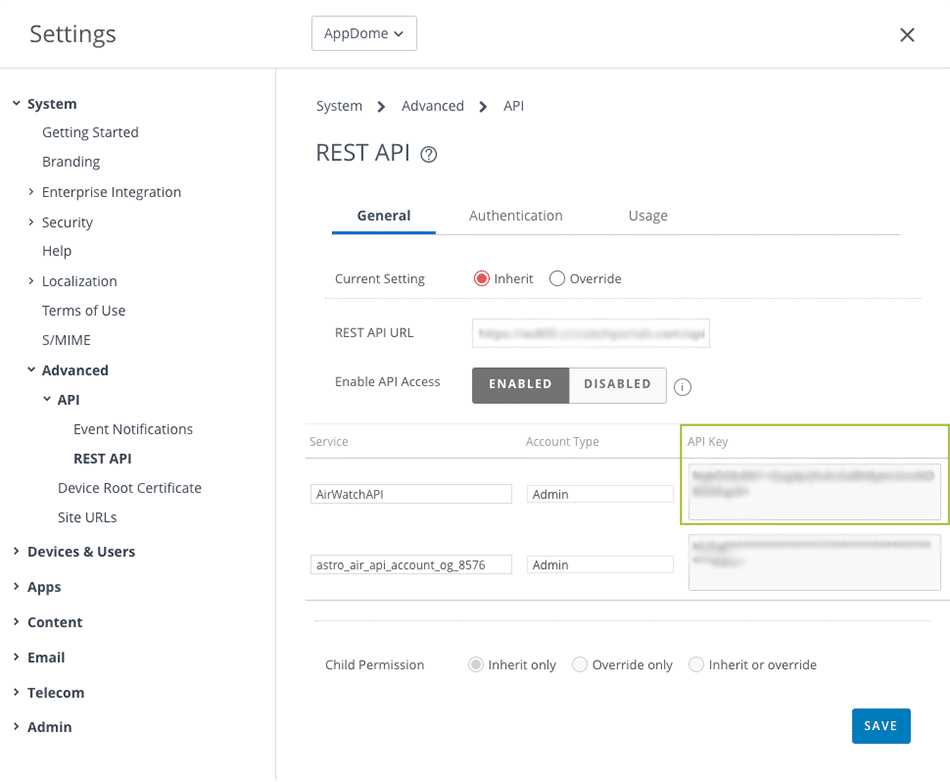A detailed caption for the described image is provided below:

---

**Image Description: Detailed Settings Menu in AppDome Application**

This image is a detailed screenshot of the settings menu in an application named "AppDome". The menu features various configurable options under the "System" settings, specifically focusing on the REST API settings.

- At the top of the screenshot, the hierarchical navigation shows "System" followed by an arrow pointing to "Advanced".
- Below this, prominently titled in capital letters, is "REST API".
- An underline and highlighted text "General" mark the current sub-menu, with "Authentication" and "Usage" also listed but not highlighted.
- Under the general settings, "Current Setting" shows two options labeled "Inherit" and "Override", represented by clickable circles. The "Inherit" option is selected, indicated by a red-filled circle.
- Following this, the text "REST API URL" is displayed, adjacent to a text box containing a blurred-out URL.
- Next, the setting "Enable API Access" is presented with a switch toggle that is set to "Enabled" and highlighted in gray.
- The "Service Account Type" section has "API Key" selected, emphasized by a green square around it. The actual API key in a nearby text box is blurred out.
- Towards the bottom, "Child Permission" configurations are presented with options for "Inherit Only", "Override Only", and "Inherit or Override". "Inherit Only" is chosen but grayed out, indicating it as a fixed or default setting.
- At the bottom right corner of the image, there is a "Save" button for confirming changes to the settings.

To the left side of the image, there are additional menu options under the "Settings Menu". Listed under "System" are options such as "Getting Started", "Branding", "Enterprise Integration", "Security", "Help", "Localization", "Terms of Use", and "S/MIME". Bold text highlights sections under "Advanced", including "API Event Notifications", "REST API", "Device Root Certificate", "Site URLs", "Device and Users", "Apps Content", "Email", "Telecom", and "Admin".